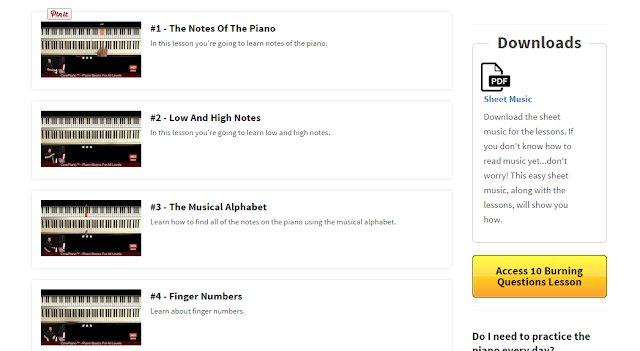This image is a screenshot from a piano tutorial website. On the left side, there are four horizontally lined-up video thumbnails, each showing an overhead view of hands playing piano keys. Each video thumbnail is accompanied by a title and description: the first is "The Notes of the Piano," the second is "Low and High Notes," the third is "The Musical Alphabet," and the fourth is "Finger Numbers." 

On the right side of the screenshot, there is a section dedicated to downloading sheet music in PDF format. It includes a descriptive note reassuring beginners that even if they cannot read music yet, the easy sheet music will guide them through the lessons. Below this description is a prominent yellow rectangular button with the text "Access 10 Burning Questions Lesson."

The entire site features an all-white background, emphasizing its focus on piano tutorials.